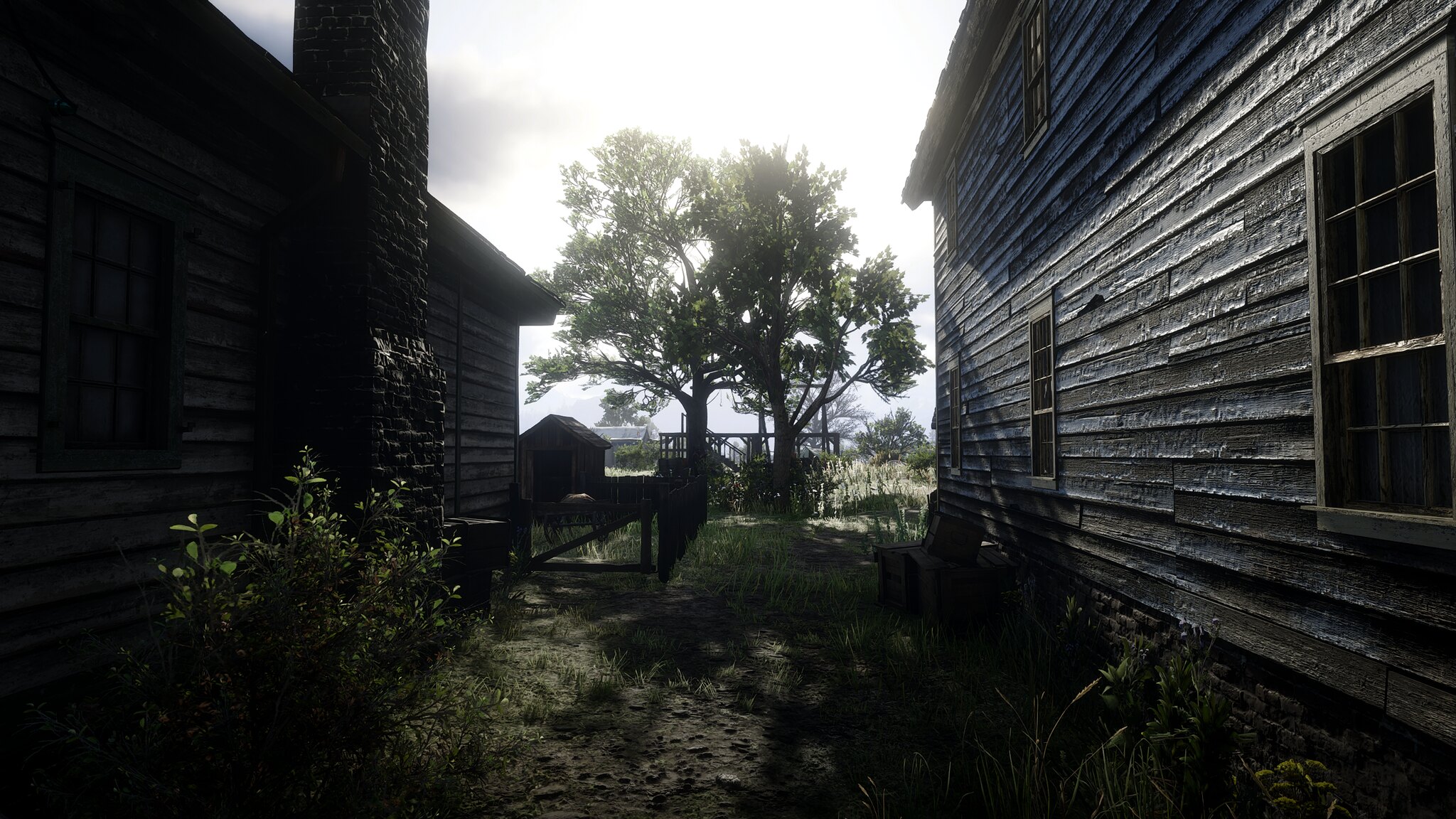In this picturesque scene, the image captures what appears to be an early morning or late afternoon setting, characterized by a soft, warm sunlight filtering through the top middle portion of the frame. The sun is partially obscured by twin trees, whose branches are adorned with a moderate but not overly dense array of leaves. Below, a patch of grass forms the central focus, with two dark grey wooden cabins flanking either side of the image. The cabin on the left features a chimney and faintly visible windows, whereas the more illuminated cabin on the right boasts three windows, suggesting it has two floors due to the window on the second level. In the middle ground, slightly off-center, there is a small, somewhat dimly lit dog house, adding a charming touch to the rustic atmosphere.